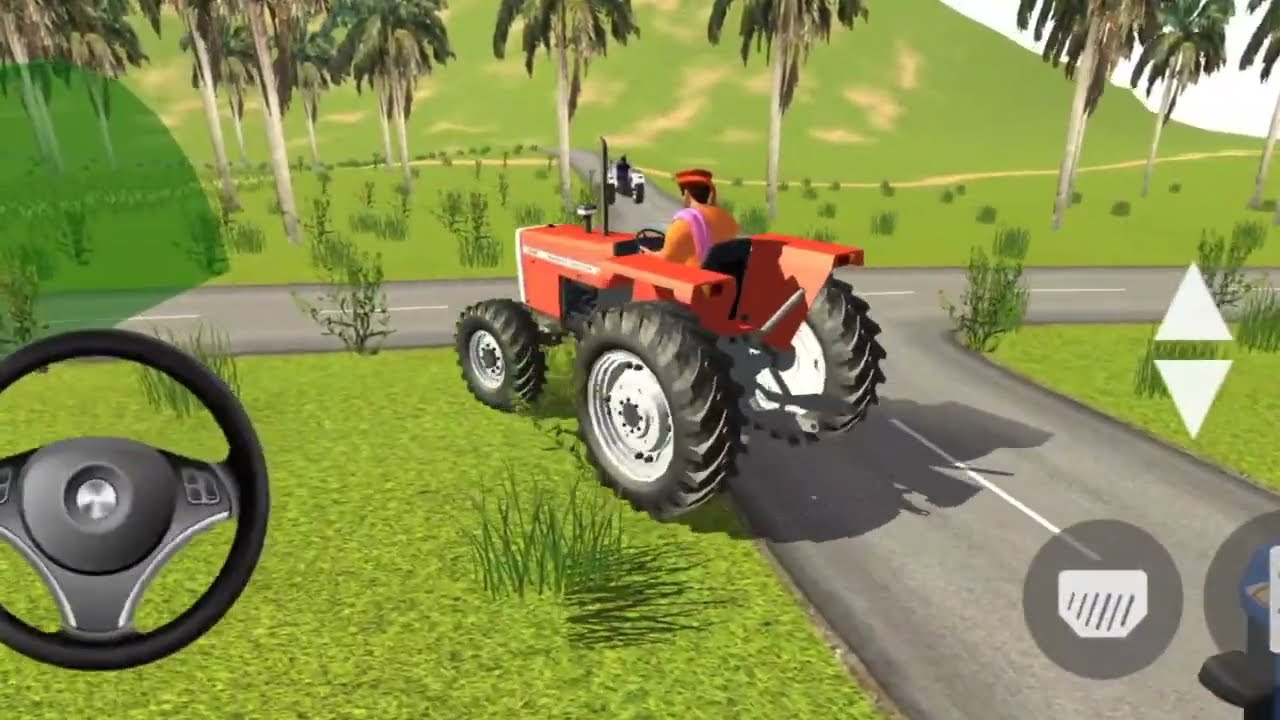The image appears to be a screenshot from a mobile or computer simulation game, depicting a brightly animated farm scene. Central to the image is a large red tractor with two enormous rear wheels and smaller front wheels, driven by a character dressed in an orange top, red hat, and a lavender cloth draped over his left shoulder. The tractor is partially off the road, moving onto the grass of the lush, green landscape. The left side features an on-screen steering wheel control panel, while the right side shows directional arrows (up and down) along with additional symbols and what appears to be a brake pedal. In the background, there's a winding road, green hillside, palm trees, and bushes, all under a clear, sunny sky, as indicated by the shadow cast by the tractor.